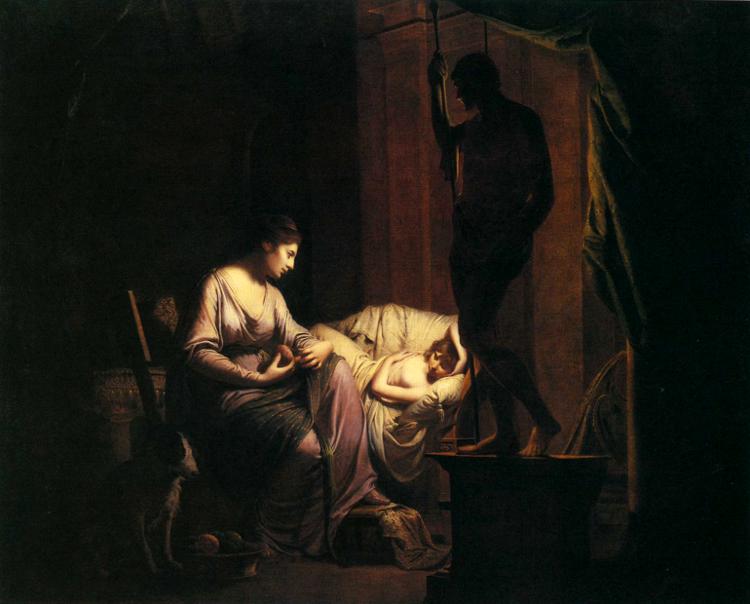The painting depicts an old, Renaissance-style scene with a dramatic interplay of light and shadow. The background is entirely black, casting the central figures into striking relief. On the left-hand side, a woman with dark, tied-back hair radiates a soft, illuminating light that highlights her worried features. She is draped in a loose, purple garment reminiscent of a shawl, sitting gracefully on a chair or couch. Next to her lies a child, possibly a girl, topless and covered partially by a white sheet. The child appears to be reclining with an arm across their chest, evoking a sense of vulnerability. To the right, shrouded in darkness, is the black silhouette of a man, his form barely discernible save for his outline and the sense that he might be unclothed. Nearby, in the shadowy background, a dog sits beside a bowl, partially hidden by the encompassing darkness. The overall mood of the painting is somber, with a palpable tension in the air, underscored by the woman's anxious gaze toward the child.